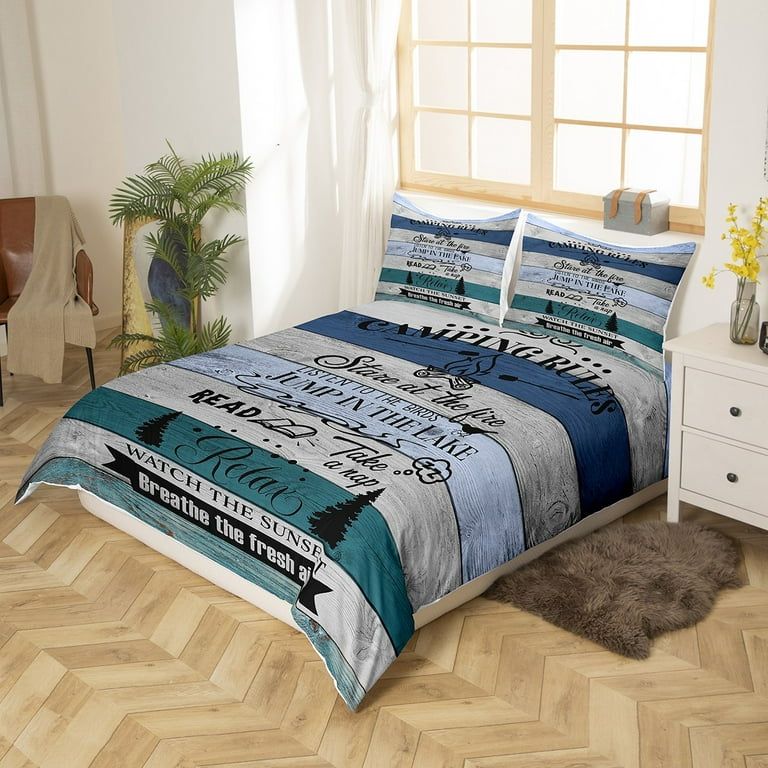The image depicts a well-arranged bedroom with a paneled wood floor and a white wall. Dominating the scene is a bed featuring a comforter and pillows with a unique pattern of wide stripes in alternating shades of gray and blue. Both the comforter and pillows are adorned with various printed phrases in black text, themed around "camping rules." These include "stare at the fire" accompanied by a campfire illustration with marshmallows on sticks, "listen to the birds," "jump in a lake," "read" with an image of an open book, "take a nap," "relax," "watch the sunset," and "breathe in fresh air." To the right of the bed stands a white dresser with two drawers, topped with a bouquet of sparsely decorated yellow flowers. Additionally, there's a thin wooden window and a small white end table with black handles on the right side. A small leather chair draped with a brown blanket and a black fur rug add further comfort to the room. The overall ambiance emphasizes relaxation and a love for the outdoors, making the bed the central focus of the picture.